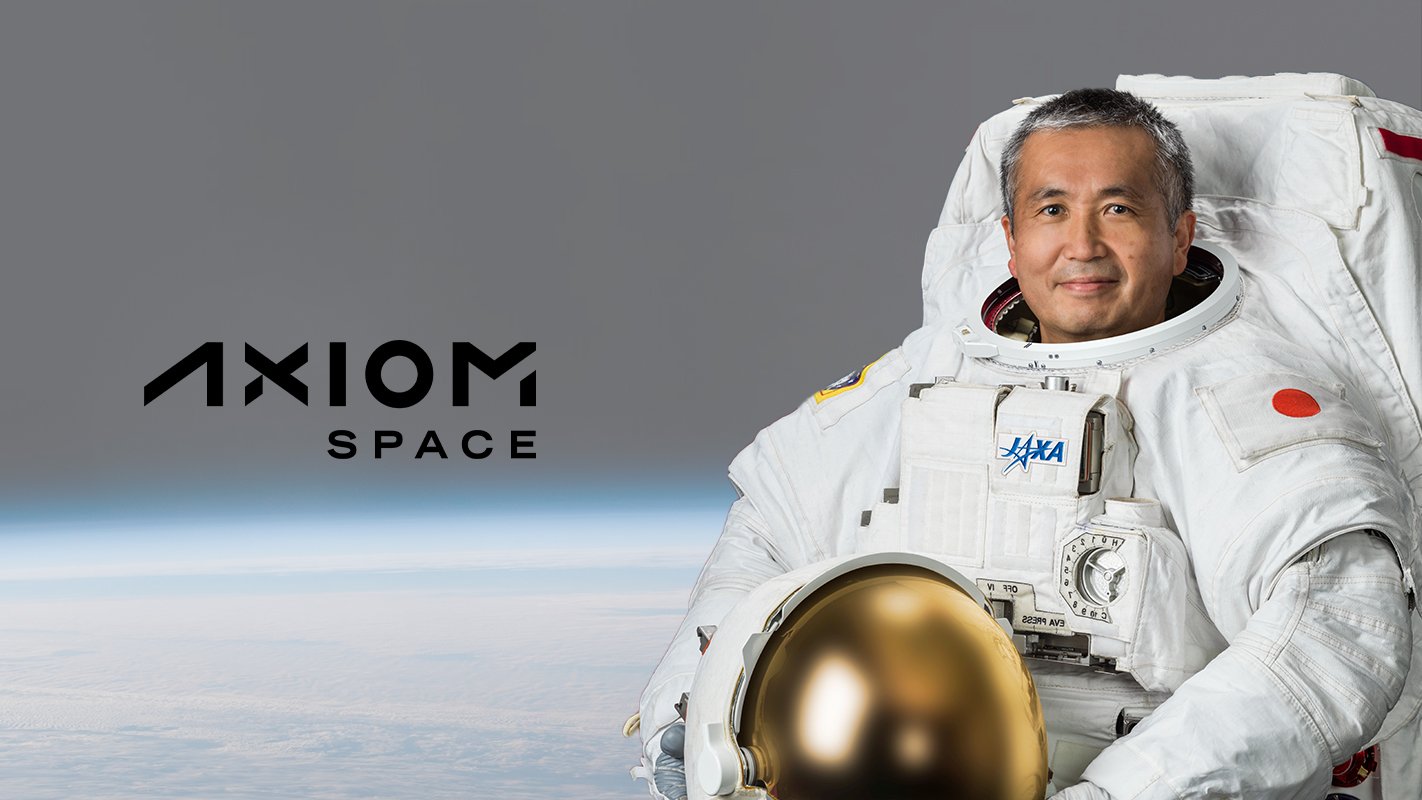The image features a portrait of an older Asian man, wearing a large, puffy white spacesuit branded with "JAXA" in blue writing on the front. The suit includes various patches, including a Japanese flag on the left arm and an additional patch that is slightly out of focus on the other shoulder. He has graying, salt-and-pepper hair and fine lines and wrinkles, giving him a distinguished appearance. His expression is pleasant, with a faint smile that doesn't reveal his teeth. In his hand, he holds a helmet with a gold visor and a white backing. To the left of the man, the brand name "Axiom Space" is prominently displayed in black, with "Axiom" written in a modern font featuring slits, and "Space" in a simpler, smaller font underneath. The background simulates outer space, with a blurred, expansive black sky and the faint horizon line of a flat, blue planet-like structure, presumably Earth, taking up about the bottom third of the image. The entire setup gives the impression of an advertisement, potentially for a flight company.